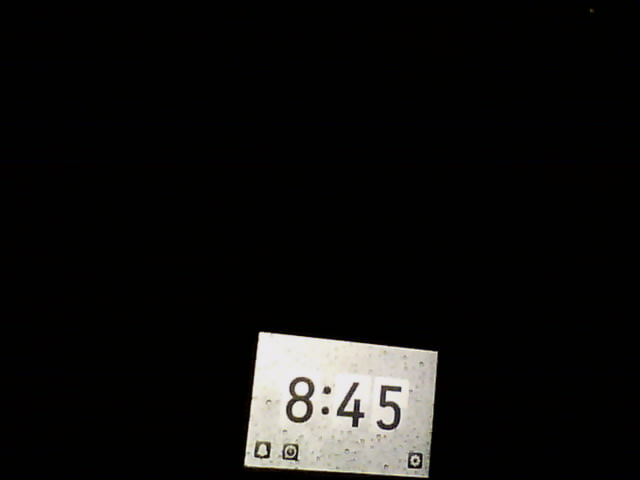The image features a digital screen that is likely part of a car's dashboard, given its shape and layout. Dominating the center of the screen is the time display, which reads "8:45" in bold black text against a white background peppered with numerous black dots. Along the bottom of the screen are a series of icons: two on the left and a third on the right, separated by a significant gap in the middle. The leftmost icon resembles a bell, indicative of notifications or alerts, and is styled in white against a black background. Next to it is an icon of a clock, similarly colored white on a black background. On the far right, there is another icon that appears to be an alarm clock, also white on a black background. The rest of the screen around these elements is entirely black, emphasizing the central time display and the icons at the bottom.